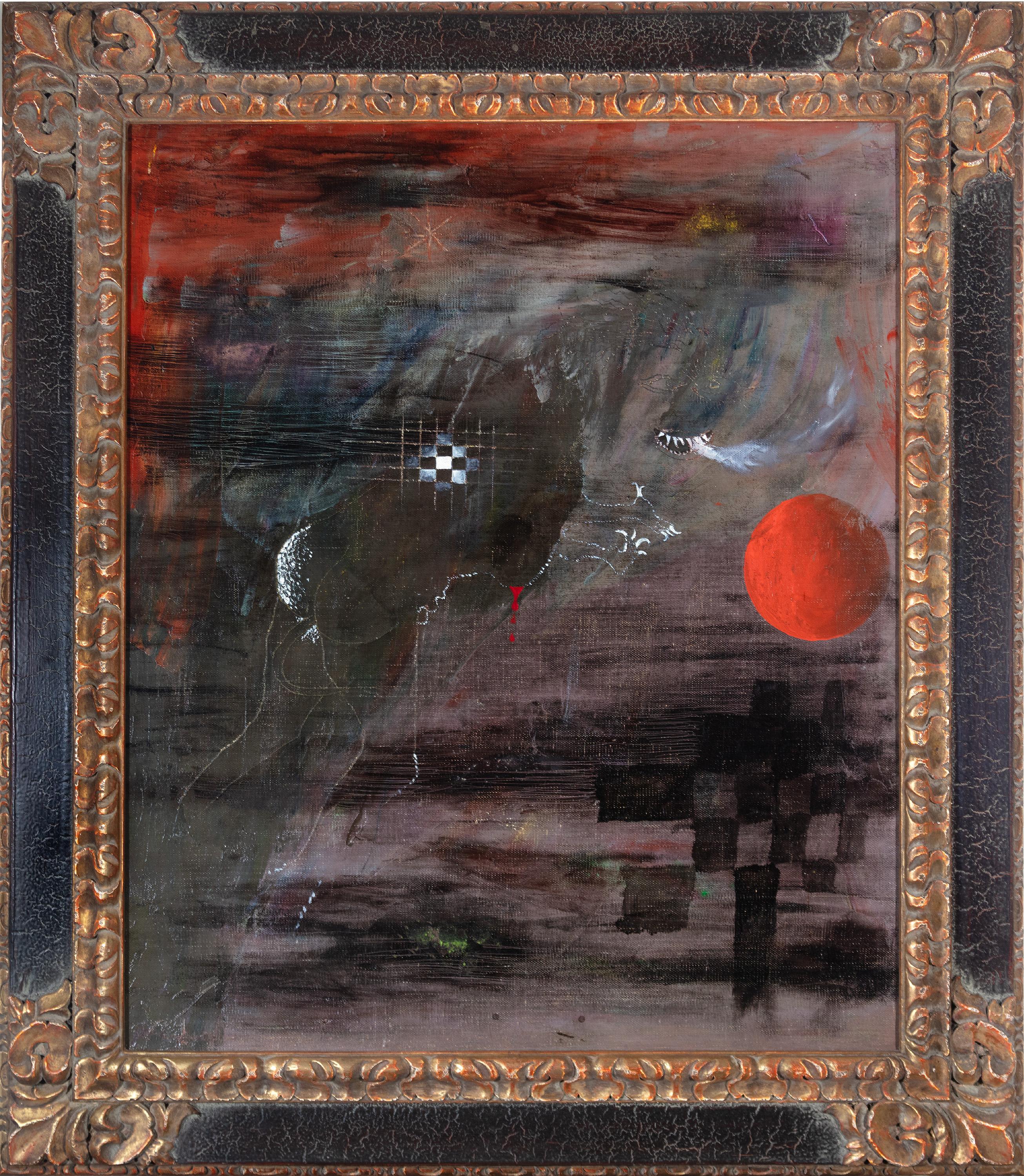The painting, encased in a meticulously ornate gold frame adorned with intricate fleur-de-lis on its corners, presents a surreal and abstract scene that merges natural and nightmarish elements. The frame’s outer border is black, possibly textured leather, which adds to its aged and weathered look.

Dominated by dark hues and sparse bright colors, the painting features a dramatic waterfall cascading over a cliff, interspersed with peculiar elements such as black and white checkered patterns, floating clouds, and a single patch of green grass at the base. A striking red sphere, reminiscent of a planet or sun, appears to the side, contrasting starkly against the otherwise somber palette.

Further adding to the surrealism, a grotesque mouth with sharp, fanged teeth is integrated into the waterfall, exhaling a ghostly white mist. The presence of a sinister “nightmare creature” with many fangs, enveloped by a blood mist, stares hauntingly, seemingly breathing hellish fire. This unsettling figure, along with the eerie moon positioned halfway down the cliff, enhances the painting’s otherworldly and disturbing atmosphere. Various textures suggest the use of charcoal or finger smudges for certain fine details, deepening the intricate and layered feel of the piece.